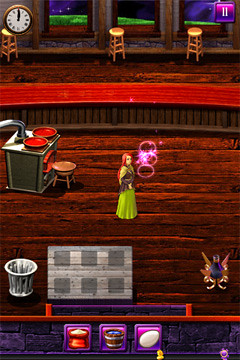In this screenshot from an older video game, a lady with long red hair is prominently featured, wearing a green dress. She appears to be casting or interacting with three pink circles adorned with stars in front of her. Behind her stands a silver stove with a pipe extending upward, flanked by two red bowls placed on top. A small wooden stool sits in front of the stove. Below this, a red line divides the scene, with a bag of flour, a barrel of water, and an egg visible at the bottom portion of the image.

The background reveals a well-detailed kitchen interior with a clock showing 12 o'clock. Three windows line the wall, each accompanied by wooden bar stools. The floor is recessed, adding depth to the space. To the left, a trash can is situated beside a table holding four gray squares. On the right, a discernible symbol adds to the game's immersive environment.